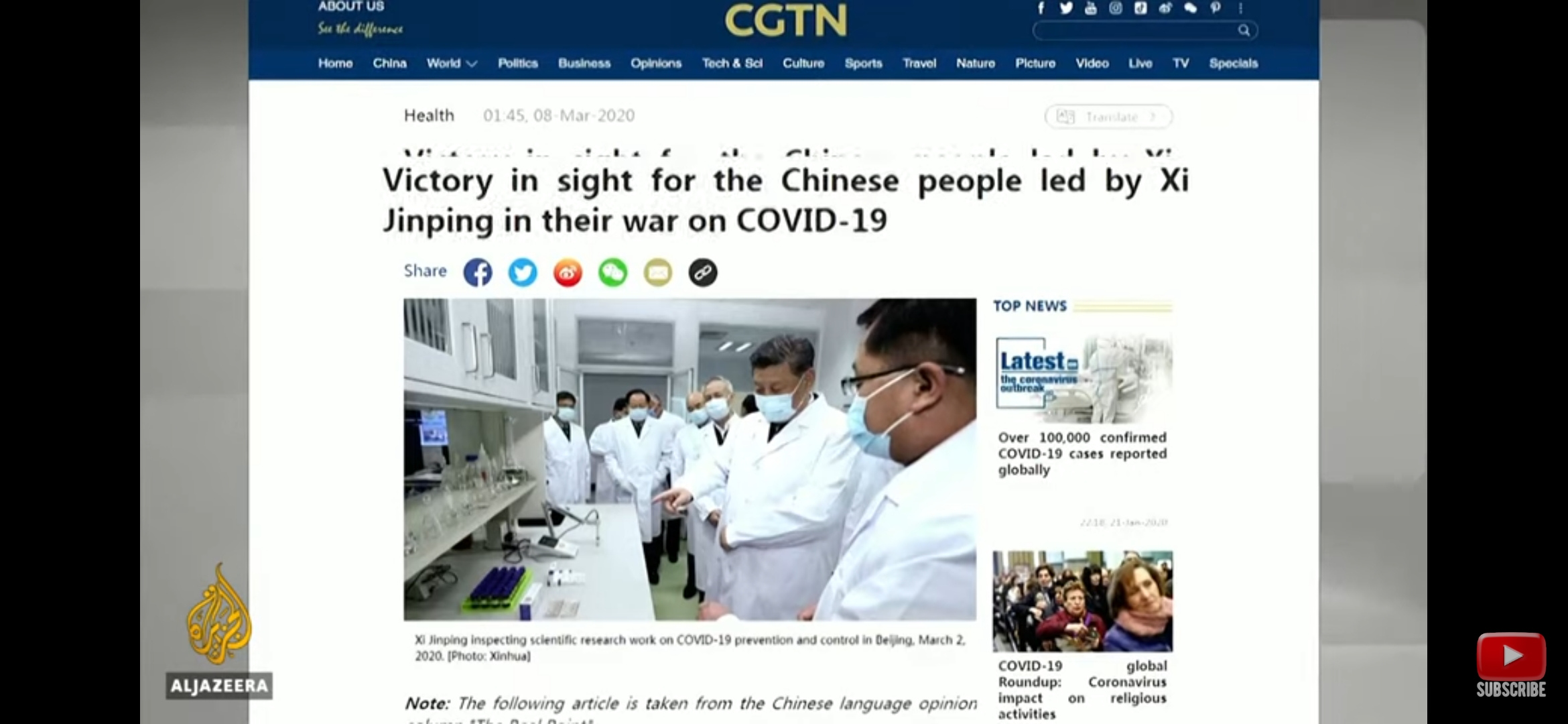The caption below refines and organizes the provided description into a detailed summary of the image:

---

The screenshot depicts the homepage of CGTN (China Global Television Network), distinguished by its large, gold-colored "CGTN" logo prominently displayed at the top right, alongside various social media icons such as Facebook and Twitter. To the left, in the top left corner, is the "ABOUT US" link, written in all white capital letters with the slogan "See the Difference" below it in a handwritten cursive yellow font. 

The navigation bar beneath offers numerous options: Home, China, World (with a drop-down menu), Politics, Business, Opinion, Tech & Sci, Culture, Sports, Travel, Nature, Pictures, Video, Live, Teaching, and Specials.

Featured beneath this navigation bar is an image of a group of scientists, clad in white lab coats and face masks, gathered around a specimen on a white table. The caption beneath the image reads, "Xi Jinping inspecting scientific research working on COVID-19 prevention from March 2, 2020." The image suggests a scene in China, with approximately six individuals pointing at the specimen.

Above the image, a bold headline proclaims "Victory in sight for the Chinese people led by Xi Jinping in the war on COVID-19." To the right, there are options to share the content via Facebook, Twitter, and other social media platforms.

The "Top News" section to the right highlights significant updates, including over 100,000 confirmed COVID-19 cases globally, illustrated with an image of anxious individuals sitting outdoors. Another story discusses the impact of COVID-19 on religious activities worldwide.

---

This caption provides a structured and enriched description, enhancing the clarity and completeness of the image's content.